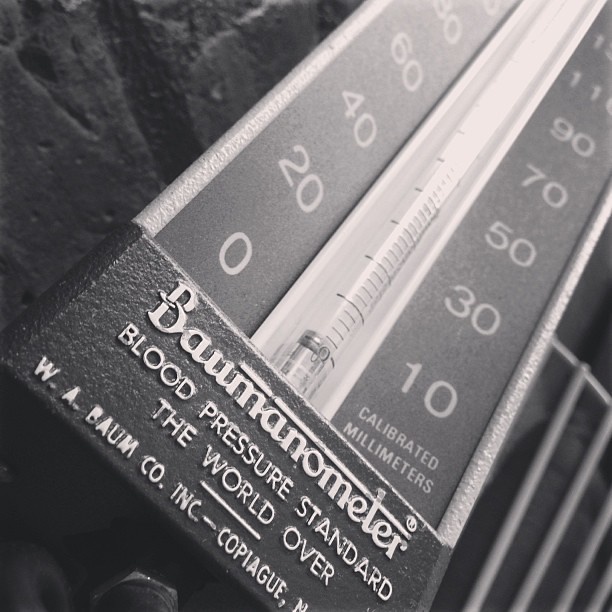The black and white image showcases a Baumanometer blood pressure monitor in a close-up shot. We are viewing the device from an oblique angle, focusing predominantly on the bottom section where the brand name and manufacturing details are located. The photograph clearly displays the brand “Baumanometer” (registered trademark) along with the slogan, "Blood Pressure Standard the World Over." Additionally, it features the manufacturer's details: "W.A. Baum Company, Incorporated, Copiag," with the remaining location slightly cut off, likely indicating New York or New Jersey.

In the foreground, a glass tube filled with mercury is visible, marked with the scale labeled in calibrated millimeters. The scale reads from zero up to about 110, with the numbers alternating on either side of the mercury column. At the zero mark on the scale, we can observe a small amount of mercury. The focus of the image is sharpest around the brand name and the glass tube.